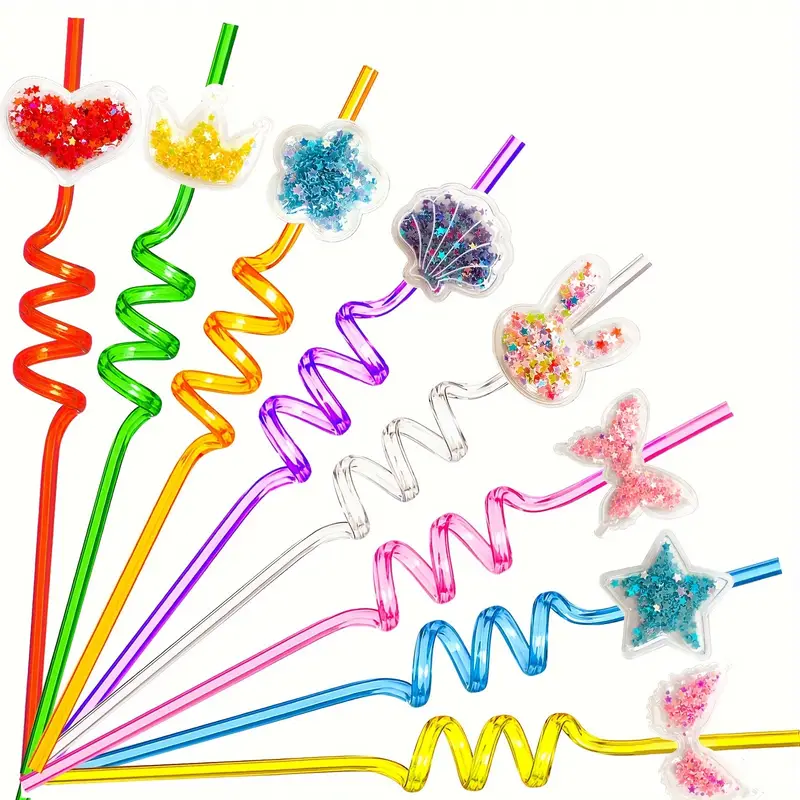This vibrant color photograph showcases an array of eight playful silly straws, elegantly fanned out from the bottom left corner of the frame. Each straw is adorned with a uniquely charming decoration, as follows:

1. The first straw on the far left is a striking red, featuring a clear heart at the tip, filled with shimmering red star-shaped glitter.
2. Next is a green straw, adorned with a clear crown filled with glimmering gold star-shaped glitter.
3. The third straw is bright orange, boasting a clear flower decoration brimming with dazzling blue star-shaped glitter.
4. Following is a purple straw, with a clear shell decoration containing multicolored star-shaped glitter that sparkles in the light.
5. The fifth straw is transparent, highlighting a cute bunny head filled with a rainbow of star-shaped glitter.
6. A pink straw comes next, decorated with an elegant butterfly, filled with shimmering pink star-shaped glitter.
7. The penultimate straw is a cool blue, featuring a striking star decoration filled with turquoise star-shaped glitter.
8. Finally, a cheerful yellow straw completes the arrangement, adorned with a clear bow filled with radiant pink star-shaped glitter.

Together, these whimsical straws create a visually captivating and festive display.